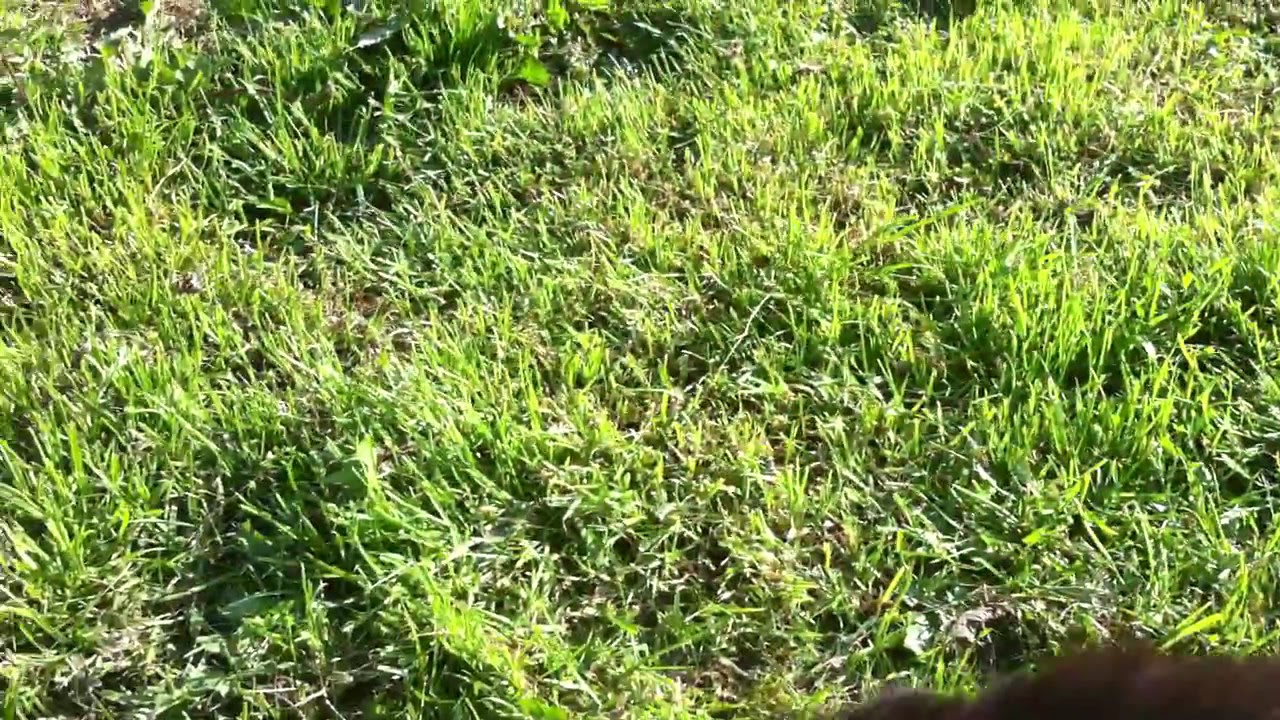The image features a lush, green lawn captured from a first-person perspective, pointing straight down. The vivid green hues dominate the scene, suggesting the grass is both healthy and natural. Although it is mostly a bright, vibrant green, there are occasional hints of brown scattered throughout, indicating a few patches where the grass might be drier or less manicured.

The grass appears somewhat overgrown, giving an impression that it might need a trim soon. There are some weeds interspersed among the grass blades, adding to the naturalistic feel of the setting. The sunlight, indicative of a mid-summer day, casts a warm glow over the lawn, enhancing the green vibrancy.

In the lower right corner of the image, there’s a slightly blurred area that might be part of the photographer’s arm or leg, suggesting their presence in the shot. This blurred portion is minimal but noticeable, slightly disrupting the otherwise uniform view of the grass. The grass blades extend throughout the entire frame, indicating that the photo was taken simply by pointing the camera downwards, possibly in a backyard, a park, or another well-kept outdoor space.